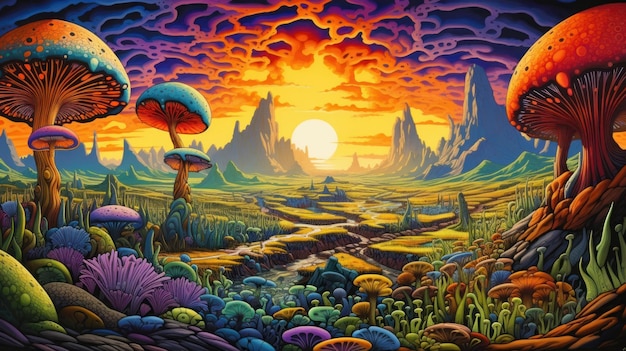This vibrant, surreal painting captures a psychedelic landscape dominated by giant, fantastically designed mushrooms. The mushrooms, in an array of colors including red, blue, green, and yellow, start from the bottom of the image, with some towering on both sides. A prominent blue mushroom stands slightly off-center. In the background, the scene is lit by a sun that's almost fully visible, except for its bottom left part, which is obscured by jagged, sharp-pointed mountains. Additional mountain peaks of various sizes stretch to the right of the sun. The sky is ablaze with vivid oranges and purples, filled with squiggly, almost cloud-like patterns. The overall setting suggests either a sunrise or sunset, casting a golden hue across the fantastical landscape, where surreal purple plants and gold and green valleys further enhance the dreamlike atmosphere.